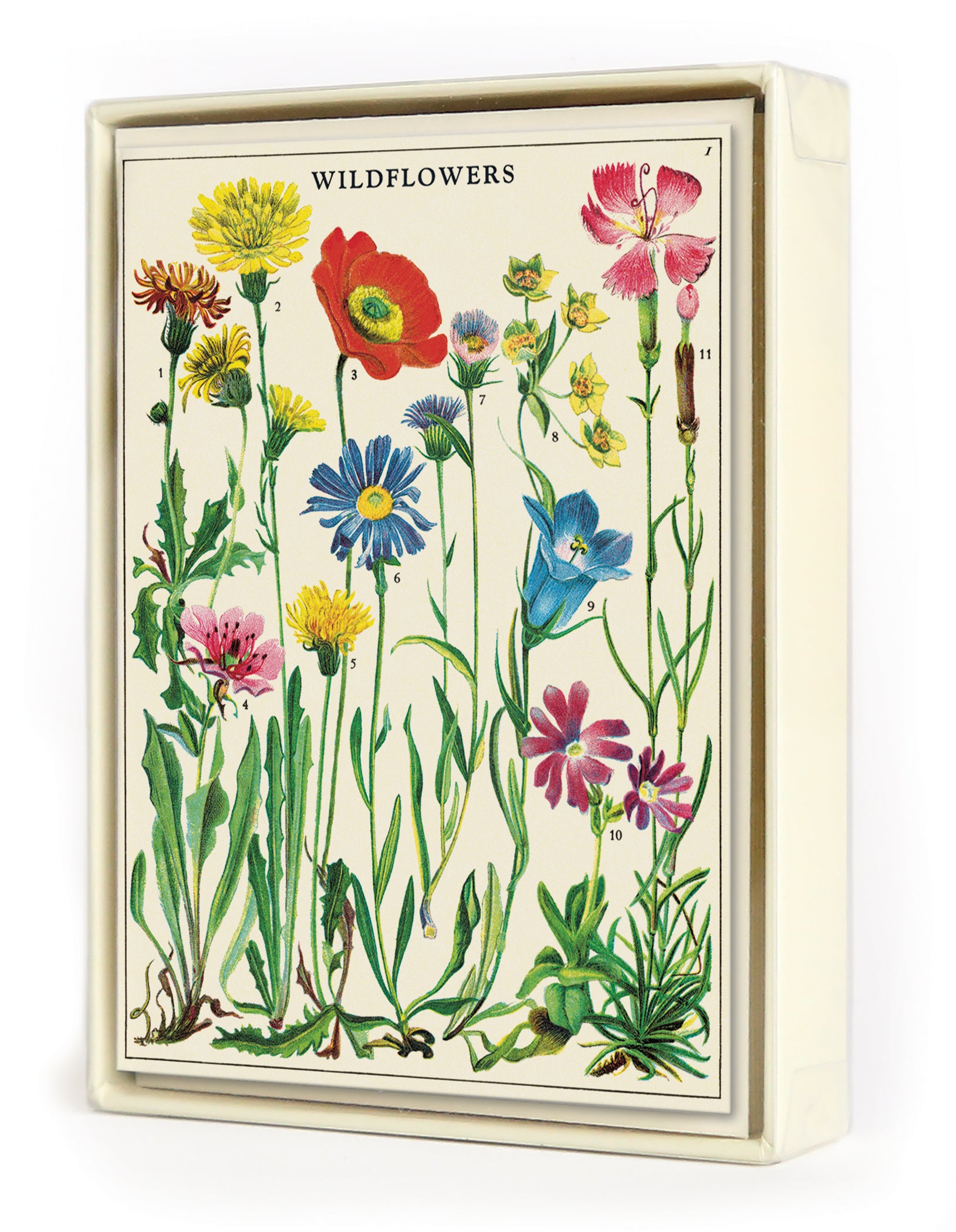The image portrays a vertically aligned rectangular picture, possibly a photo of a framed painting, mounted on a white backdrop. The setting appears to be indoors. The picture has an ivory-colored border with a thinner, dark brown or red inner border. At the top, the title "WILDFLOWERS" is prominently displayed in all caps black letters. The artwork features a collection of vibrant wildflowers with green stems, arranged vertically and tall. The flowers are meticulously numbered and include an array of colors: pink on the left, three yellow flowers paired with a pink one in the top right corner, followed by a red flower with a yellow center to the right. Below is a blue flower with a yellow center, alongside a lineup of yellow, blue bulb-shaped, and five smaller yellow flowers. Further to the right, there is a large pink flower, and in the bottom right, violet-colored petals form another flower. The bottom section of the picture is adorned with tall, narrow green leaves and a touch of grass in the lower right corner, complementing the floral arrangement.